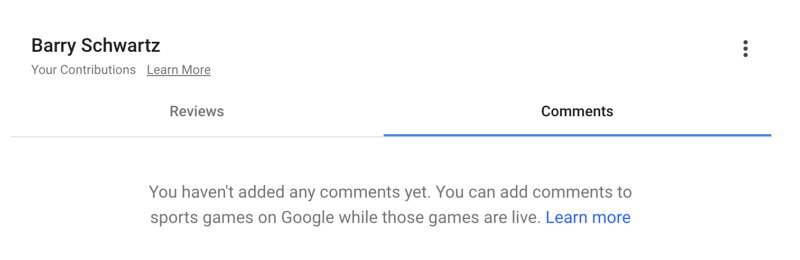This is a detailed screen capture of a website or application interface, presented within a horizontal rectangular frame. The background is predominantly plain white, accentuated with black, gray, and blue text elements.

In the upper left corner, there's bold black text reading "Barry Schwartz." Directly underneath this, in a smaller and finer gray font, it states "Your Contributions, Learn More." The upper right corner features a vertical three-dot icon, indicating a menu or settings option.

Just below this header section, a horizontal gray line spans the width of the image. Above this line, the word "Reviews" is in gray on the left side, while "Comments" appears in black on the right. The right half of this gray line is underscored with a bold blue line, highlighting the "Comments" section.

Below the blue-highlighted line, the text is displayed in a light gray, non-bold font, stating: "You Haven't Added Any Comments Yet. You can add comments to sports games on Google while those games are live." This message is divided between two lines, with "You Haven't Added Any Comments Yet. You can add comments to" on the first line, and "sports games on Google while those games are live, learn more" on the second. The phrase "Learn More" is in blue, maintaining the same size and font, and is likely a clickable link.

The image is notably minimalistic, with no additional graphics or text elements beyond those described.